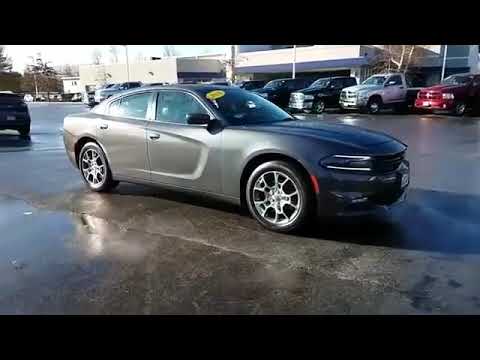The image depicts a modern Dodge Charger in a charcoal gray color, prominently placed at the center of a car dealership's parking lot. The car, viewed from a front three-quarters profile, features silver wheels and a distinctive yellow sticker on the top left of the windshield, presumed to display the price. Additionally, there is a small red strip near the front tire. The scene is brightly lit by natural daylight, underscoring the car’s shiny exterior. Surrounding the Charger, a series of pickup trucks are lined up in a row, parallel to a long, white dealership building that stretches across the background. The ground of the lot is composed of gray stone or pavement. Although no individuals are visible in the shot, the organized layout suggests an active dealership environment. Leafless trees and a faintly visible white sky indicate it might be late in the year.